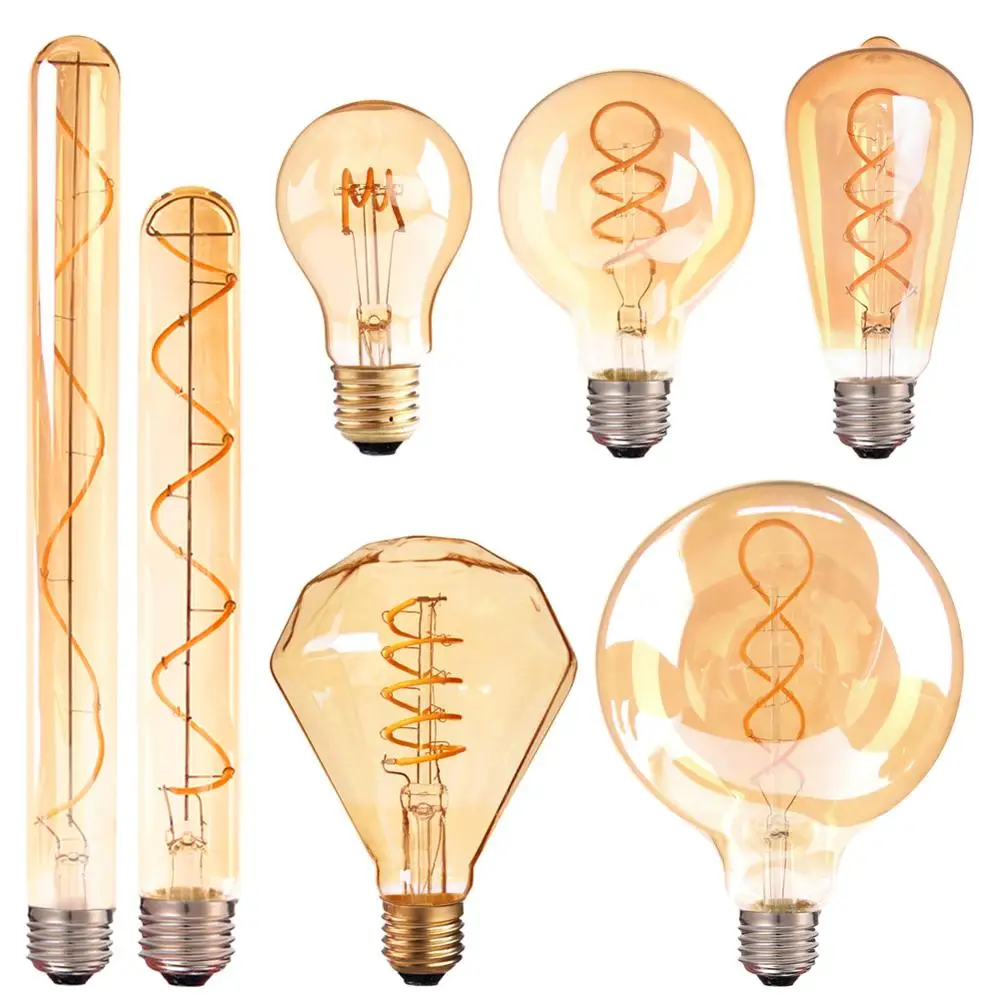The image features a collection of seven distinctive lightbulbs arrayed against a pristine white background. Each bulb boasts a unique shape and intricate filament design, demonstrating a fusion of modern complexity with a vintage amber glow. On the far left, two tall, slender bulbs catch the eye with their slight length variation and silver 826 bases; their internal filaments extend gracefully upwards. Moving right along the top row, the layout includes an almost standard-shaped bulb with an orange hue, followed by a rounder bulb with a twisted filament, and an Edison-style bulb with an oval shape and its characteristic glow. The bottom row starts with a hand-blown artisan bulb, followed by a larger circular bulb with a helix-type filament, and finally, a thick-to-thin shaped bulb. The entire collection, with its warm tones and sophisticated designs, transcends the typical lightbulb, offering a captivating aesthetic.